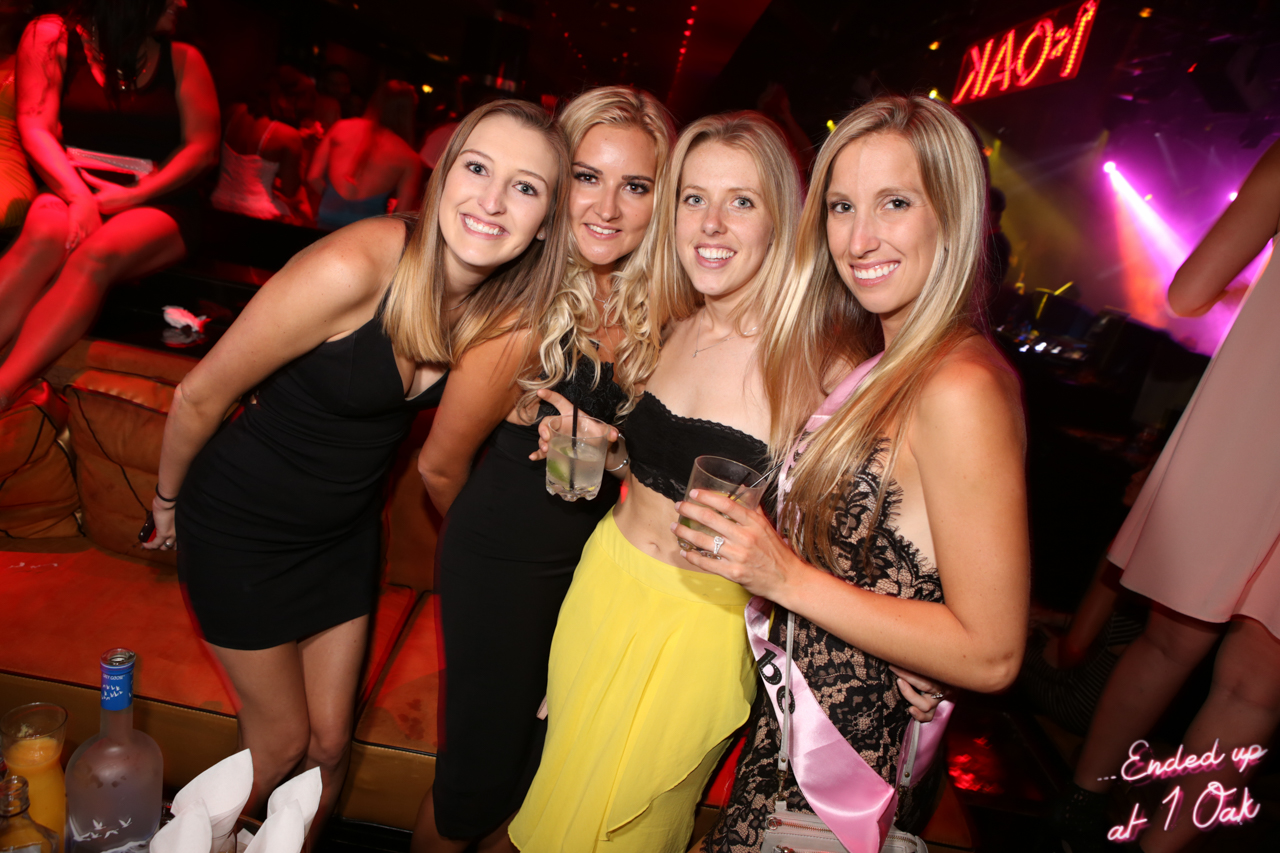The image features a vibrant nightclub scene with four young, blonde women posing at the center. All are standing and smiling, radiating youthful energy. From left to right: 

- The first woman has shoulder-length, straight blonde hair and is wearing a short black dress. She is smiling and slightly crouched towards the center. 
- To her right, another young woman also has shoulder-length blonde hair, but it starts straight and becomes curly towards the ends. She is dressed in a black dress, with her hands positioned behind her back, and she too is smiling.
- The third woman sports shoulder-length, straight blonde hair and is wearing a revealing black tube top paired with a yellow skirt. She holds a translucent drink with a lime and a black straw.
- The woman on the far right has straight, shoulder-length blonde hair, a pink sash with black writing draped across her shoulder, and is smiling as well. She holds a drink in a circular cup with a black straw, and her black, frilly dress is partially obscured by the sash.

In the background, the nightclub is alive with partygoers, especially noticeable at the top left. To the top right, a stage with purple lighting adds to the vibrant atmosphere, while red lighting casts an ambient glow over the scene. At the forefront, on the bottom left, a bottle of chilled vodka (possibly Svedka or Absolut) and a cup of orange juice are visible. The setting is punctuated by the cursive neon text at the bottom right, reading "Ended up at One Oak" in white with a pink border.